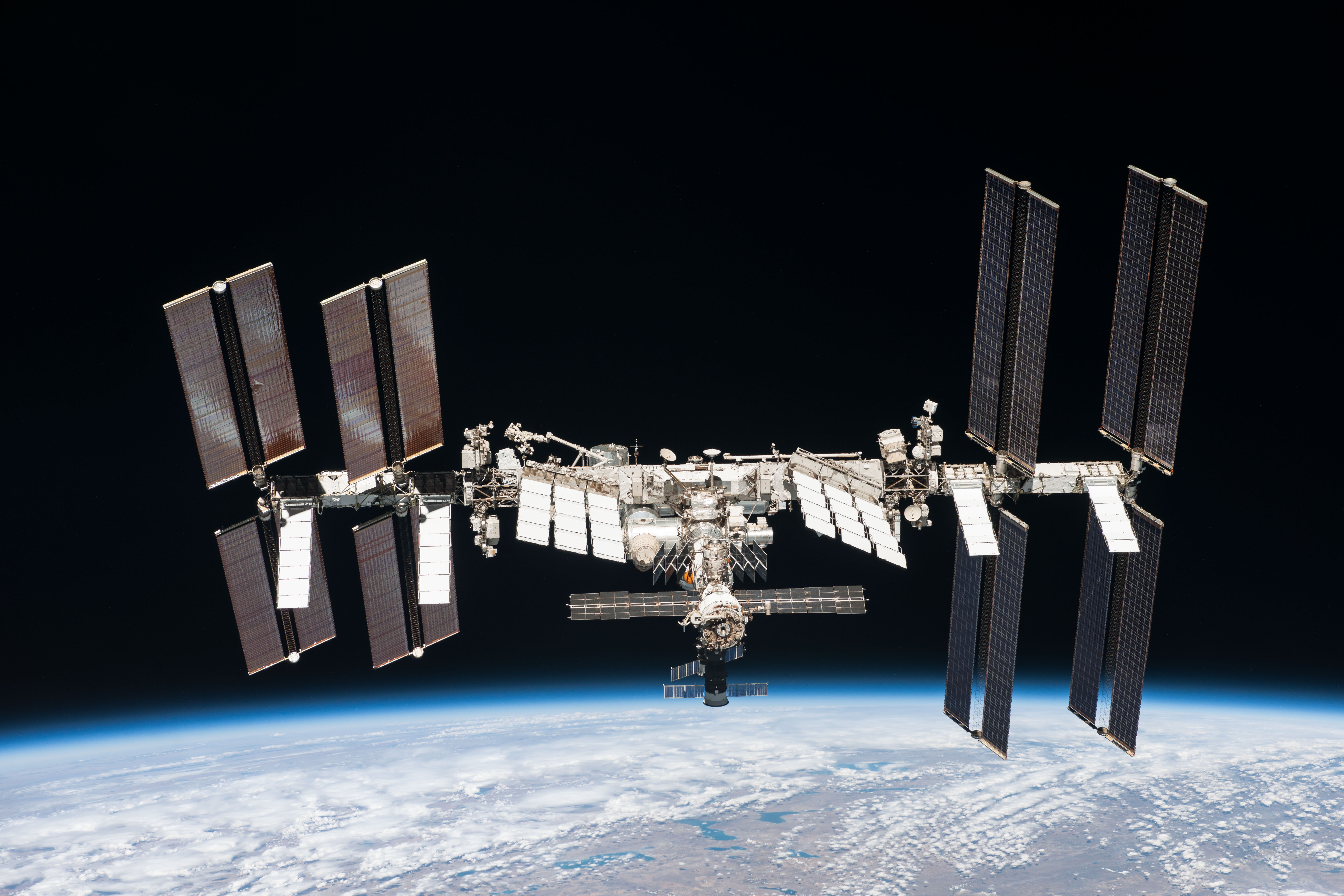The image features a high-tech satellite floating in space, captured clearly from outer space. The satellite showcases a sophisticated design with eight solar panels—organized in two symmetrical sets of four—extending from its central arms. The body of the satellite is gray, layered, and equipped with various attachments and gadgets, suggesting an intricate assembly of navigation, communication, or scientific instruments.

The backdrop of the photo is dominated by the profound blackness of space, emphasizing the isolation and technological marvel of the satellite. Approximately the bottom third of the image, however, transitions to a vibrant depiction of Earth. Here, swirling white clouds partly obscure the blue oceans and brown landmasses, while a bright light emanates from the Earth's horizon, creating a stunning corona effect that hints at the proximity of the Sun. The contrast between the dark expanse of space and the illuminated curve of Earth dramatically highlights the satellite's advanced presence in orbit.